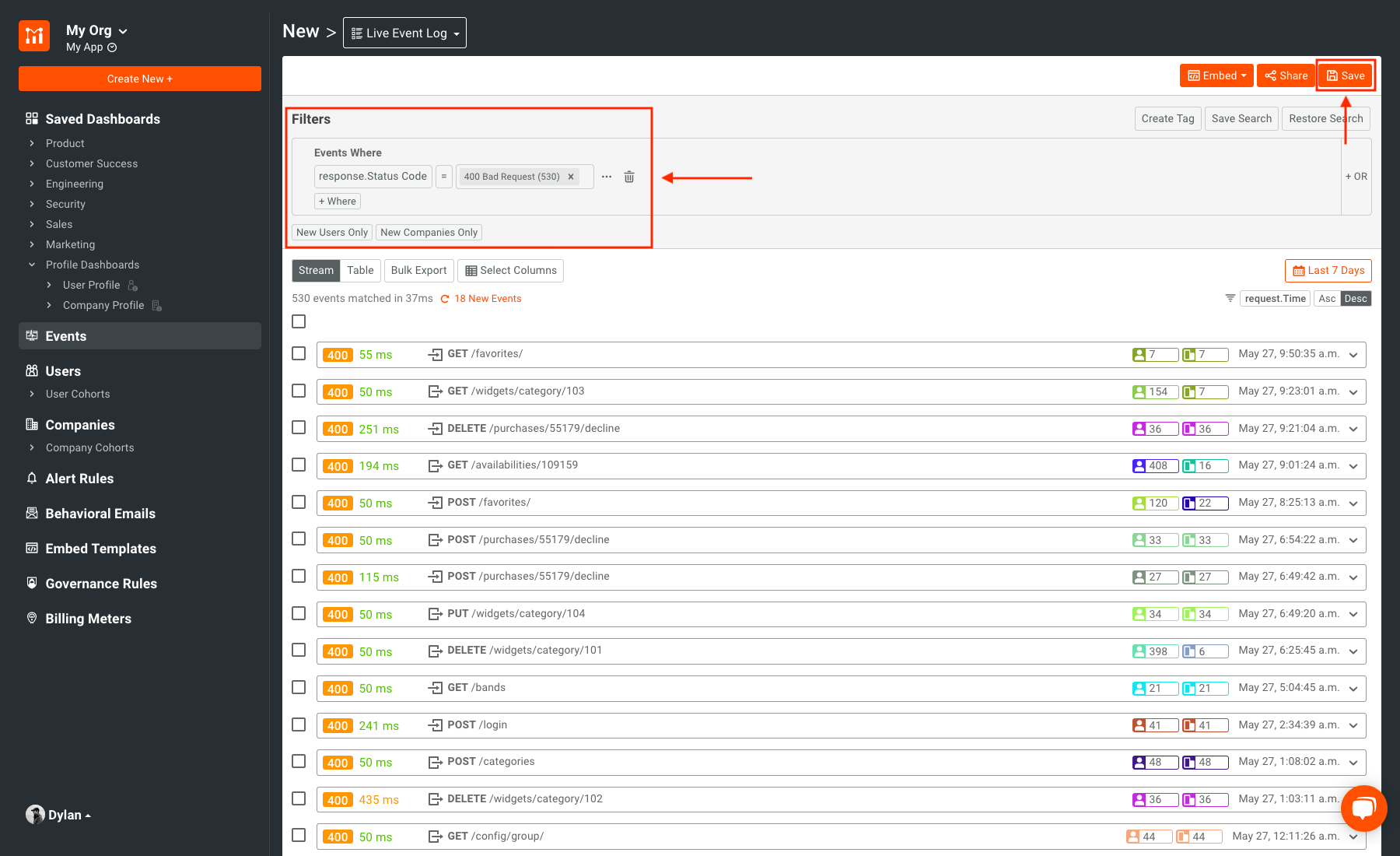### Detailed Descriptive Caption:

This screenshot captures the user interface of an application. On the left-hand side, the dark gray border features a structured menu. At the very top, labels for "My Org" and "My App" are displayed. Below them sits an orange button labeled "Create New" in white text. The menu is categorized systematically with entries such as "Saved Dashboards," "Product," "Customer Success," "Engineering," "Security," "Sales," "Marketing," "Profile Dashboards," "User Profile," "Company Profile," "Events," "Users with User Cohorts," "Companies," "Company Cohorts," "Alert Rules," "Behavioral Emails," "Embedded Templates," "Governance Rules," and "Billing Meters."

On the right side, a gray border at the top spells out "New" and "Live Event Log." Within this area, a red box highlights a section labeled "Filters." This section includes filter options such as "Events Where," "Response Status Quote 400 Bad Request," and toggles for "New Users Only" or "New Companies Only."

In the upper right-hand corner, there are three distinct orange buttons labeled "Embed," "Share," and "Save," with the "Save" button also highlighted by a red box. The interface includes additional tabs or categories named "Stream," "Table," "Bulk," "Export," and "Select Columns."

Below this, a list of events is displayed, including entries like "Get Favorites," "Get Widgets Category," "Delete Purchases 55179 Decline," "Get Availabilities," "Post Favorites," "Post Purchases 55179 Decline," "Post Purchases 55179 Decline," "Put Widgets Category 104," "Delete Widgets Category 101," "Get Bans," "Post Login," "Post Categories," "Delete Widgets Category 102," and "Get Config Group."